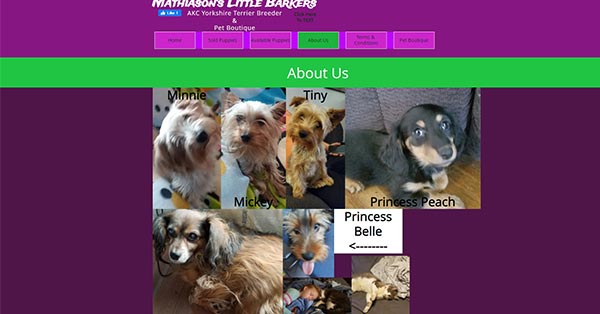A detailed description of the webpage for "Matheson's Little Bakers Yorkshire Terrier Breeder":

The webpage features a prominent violet-purple section as the background. At the top of the page, "Matheson's Little Bakers" is displayed in large text, formatted as "M A T H I A S O N apostrophe S". Below this, there is a rectangular icon with a thumbs-up symbol and the word "like" next to it, along with what appears to be the number 1, albeit slightly unclear from a distance.

In white text, the title "A X C Yorkshire Terrier Breeder" is presented boldly. The navigation bar across the top of the page contains several tabs. The first tab seems to be labeled "Home," while the second and third tabs are indistinct even when zoomed in. The selected tab is highlighted in green, contrasting with the pink and purple blend of the other tabs, which are difficult to read against the purple rectangular backdrop.

Beneath the navigation bar, another green rectangle, nearly neon but not quite, is centered with the text "About Us." 

The content then transitions to showcasing various dogs, each with their names labeled above. On the left, a Yorkshire Terrier named Minnie (spelled "M I N N I E") is featured. Next to Minnie is another Yorkie named Mikey (spelled "M I C K Y"). The following tiny Yorkie, with gold and brown fur and brown ears, is labeled "Tiny."

Additionally, a black Cocker Spaniel with brown markings on its nose, eyebrows, and feet is named "Princess Beach." Another dog appears in a white rectangle with black text indicating the name "Princess Bella" (spelled "B E L L E") and a dotted arrow pointing towards it.

The final dog showcased is a Siberian Husky, gray on top and white on its body, lying against a gray blanket and dark gray sheet. This section is set against the same violet-purple background as the rest of the webpage.